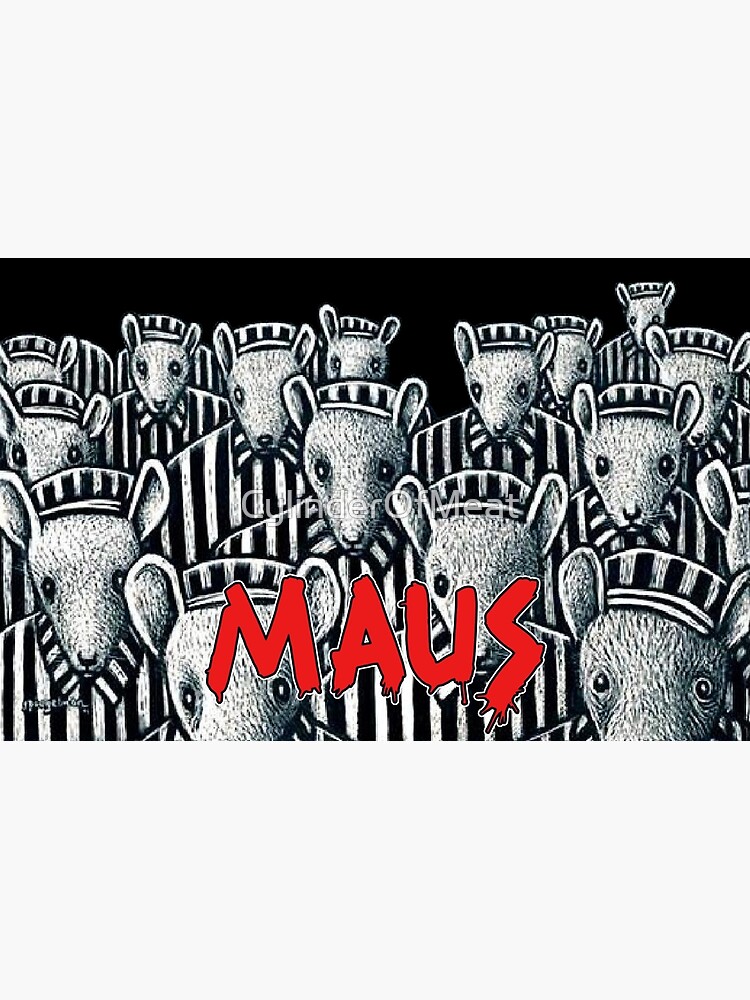The image appears to be an intricately detailed artwork resembling an album cover, portraying a multitude of humanoid mice or rats. Each figure is dressed in old-time prison uniforms, consisting of black and white striped shirts and matching hats. The haunting illustration features a dozen or more mice standing in close formation, all facing forward with dead-eyed expressions that bore into the viewer. One mouse, positioned at the bottom right, stands out with notably wider eyes, diverging from the otherwise uniform looks of the others.

Dominating the image is the striking red text "MAUS," boldly painted in a brushstroke style with drips trailing from the letters, accentuating the image’s poignant impact. The background is a solid, somber black, further amplifying the stark prison attire of the mouse characters. Subtly overlaying the center of this powerful scene is a faint watermark reading "Cylinder of Meat," just barely visible atop the group of mice. All elements drawn together provide a vividly detailed and evocative visual narrative, reminiscent of themes explored in graphic novels.